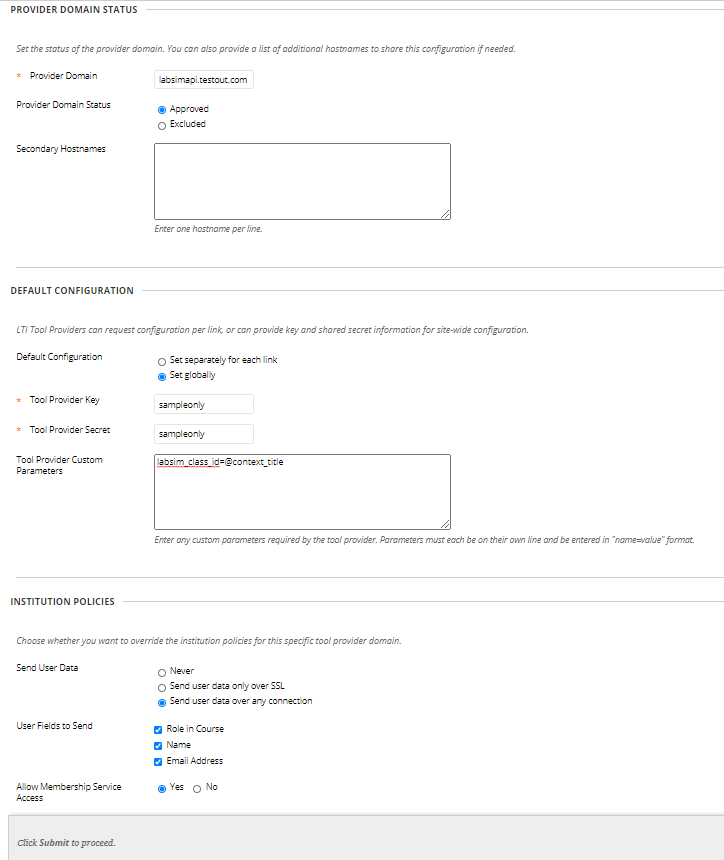The image depicts a form-like interface against a solid white background, resembling a sheet of paper. The form is divided into distinct sections, each with specific functionalities.

**First Section: Provider Domain Status**
- This section prompts the user to input their domain for status verification.
- There are interactive options to either "Approve" or "Exclude" the domain.

**Second Section: Secondary Host Names** 
- Users can add additional host names under this category.

**Third Section: Default Configuration**
- Users have the option to configure settings either separately for each link or globally.
- Fields for entering a "Tool Provider Key" and "Tool Provider Secret" are provided.
- Space for "Custom Parameters" is also available here.

**Fourth Section: Institution Policies**
- This section allows users to choose whether to override institutional policies for the specific tool or domain.
- Options are "Never" for the override.
- Includes settings for role and coordinate email addresses, as well as an option to allow membership service access with "Yes" or "No" choices.